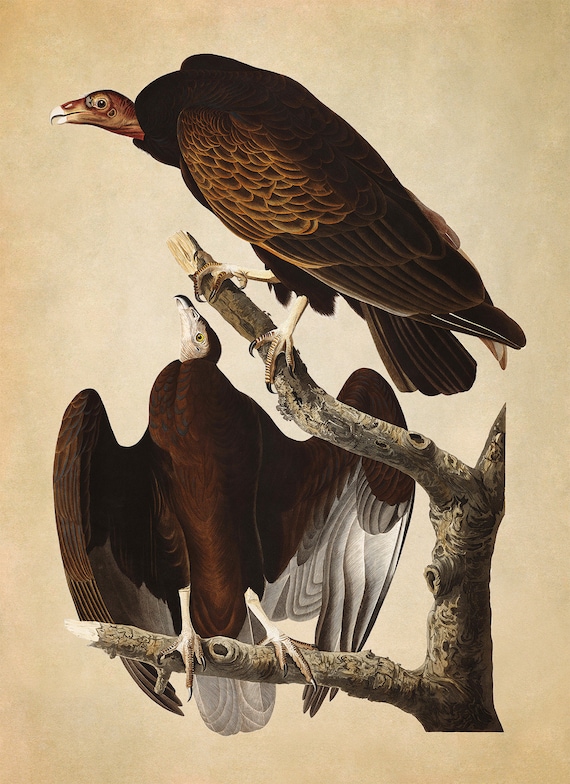In this sepia-toned photograph, two vultures are perched on the grayish-brown branches of a tree. The background features a warm, beige hue that contrasts with the birds. The vulture on the top branch is hunched with its wings down and its head tucked into its feathers, displaying predominantly brown plumage. The lower vulture, more spread out and looking up, has distinctive white markings on the underside of its wings and tail, along with a white head. The branches appear partially cut off in the image, contributing to a focused portrayal of the vultures amidst the inviting warm tones of the backdrop.